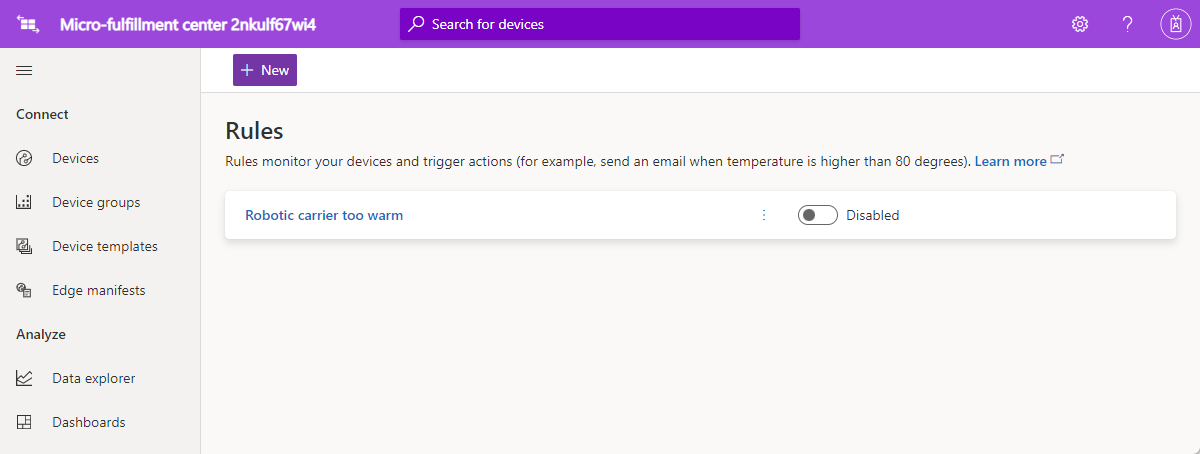A detailed screenshot captures a page from a micro-fulfillment center platform. Dominating the upper section is a wide purple bar with various elements displayed in contrasting white text. On the left side, a unique identifier "2NKULF67WI4" is prominently featured. Centrally located on this bar is a search bar with the placeholder text "Search for devices," accompanied by a microscope icon to its right. Moving further right, there are several functional icons: a gear icon representing settings, a question mark for help, and an ambiguous circular icon which may depict a stylized letter 'A' or a mobile device with antennas.

Below the purple bar, the layout transitions into a comprehensive menu system. A gray column titled "Connect" sits at the top, listing several navigation options sequentially: Devices, Device Groups, Device Templates, and Edge Manifests. Adjacent to this, another column labeled "Analyze" features subsections for Data Explorer and Dashboards, offering in-depth tools for data examination and visualization.